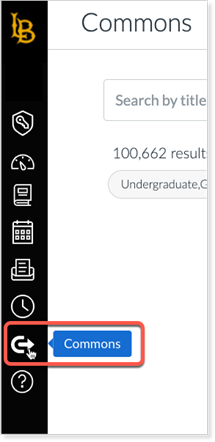In this image, we see a detailed display with multiple icons and a search interface. On the left side, at the top, there is a yellow "LB" symbol. Below this, there are eight icons arranged vertically:
1. A key within a shield
2. A speedometer
3. A book
4. A calendar
5. An envelope
6. A key
7. A clock
8. A question mark labeled "Help"

The "Commands" icon, which resembles command inputs, is selected and highlighted in either orange or red. 

To the right of these icons, the selected "Commands" section is shown in detail. At the top of this section, there is a search field labeled "Search by title" which shows 100,662 results. Below the search field, there is text displaying "undergraduates." 

The dominant colors in the image are white, black, and blue, with the selected item (Commands) appearing in a highlighted orange or red. The background behind the icons and text is black.